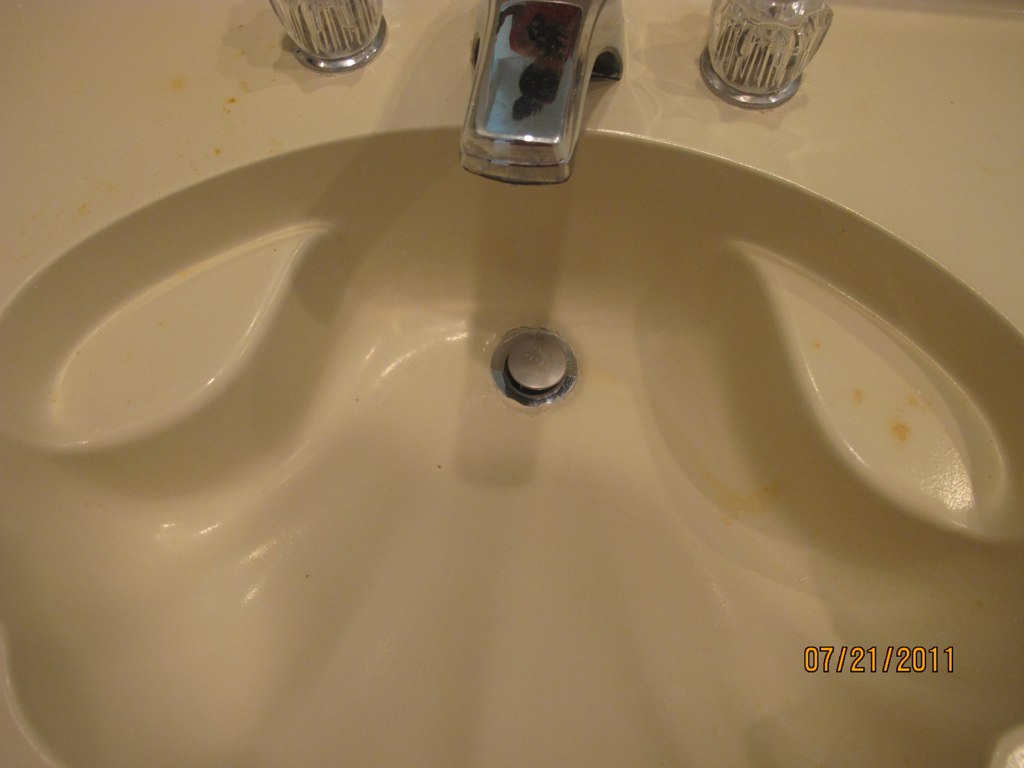The image depicts a somewhat dirty, seashell-shaped bathroom sink made of either formica, ceramic, or vinyl material. The focal point is the drain at the center, which appears dirty and in need of cleaning. The sink is white-ish and has tan, brown, and yellowish rust spots, particularly noticeable on the right side and near the left faucet handle. It features two raised platforms, or ledges, on either side of the faucet, likely intended for holding soap. The faucet itself is a standard rectangular stainless steel design with some water stains, accompanied by two clear, plastic turn-style knobs for hot and cold water. Notably, some parts of the faucet and knobs are slightly cut off in the image. At the bottom of the photo, there is a date stamp reading 7-21-2011.